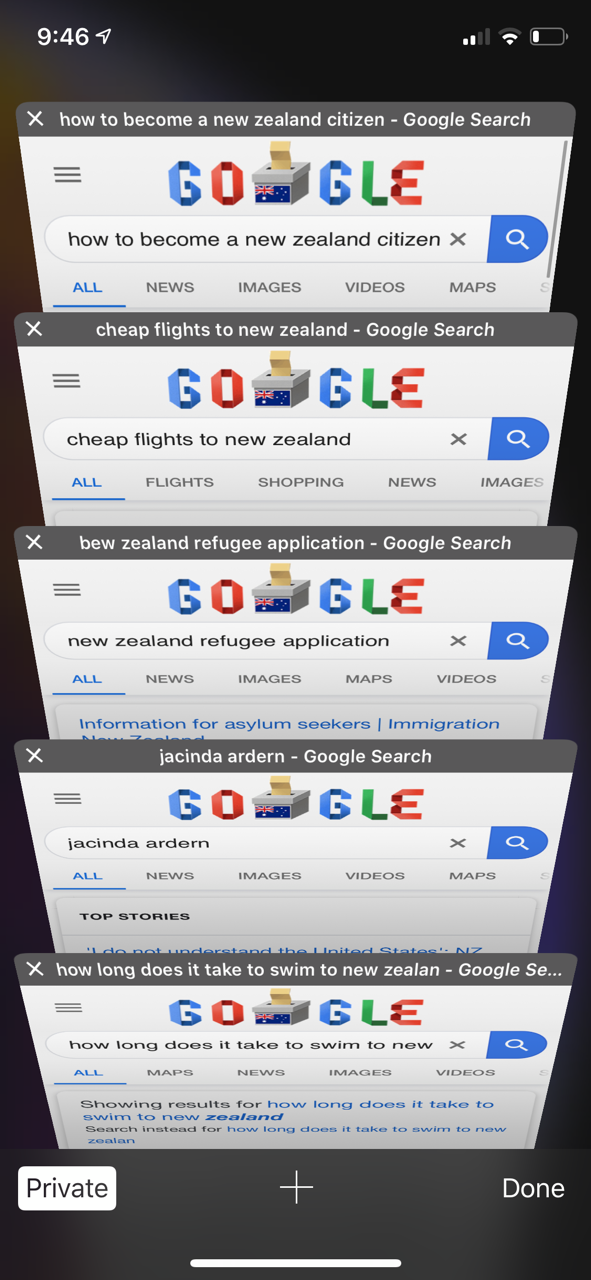The image depicts a black smartphone screen displaying various Google search results related to New Zealand, time-stamped at 9:46. The primary search bar shows a query on "how to become a New Zealand citizen," highlighted in blue and underscored, indicating an active search.

Below the main search, several boxes are present, each framed with an 'X' button in the corner for closing the individual queries. The first box contains a light blue background and three black lines followed by "Google," spelled with its iconic colored letters: a blue 'G,' a red 'O,' a stacked-papers 'O,' a blue 'G,' a green 'L,' and a red 'E.' This box also lists search categories such as News, Images, Videos, and Maps, all highlighted in blue.

Subsequent boxes include:
1. A query on "cheap flights to New Zealand," featuring similar Google categories.
2. Information regarding "New Zealand refugee application," which includes categories like "All," "News," "Images," "Maps," and "Videos" and provides details for asylum seekers and immigration.
3. A search for "Jacinda Ardern," accompanied by Google's sorting labels.
4. A whimsical query on "how long does it take to swim to New Zealand," with the standard Google search elements.

At the bottom of the image, the phone's navigation bar is black, displaying three buttons: 'Private' in white on the left, a plus sign in the center, and 'Done' on the right.